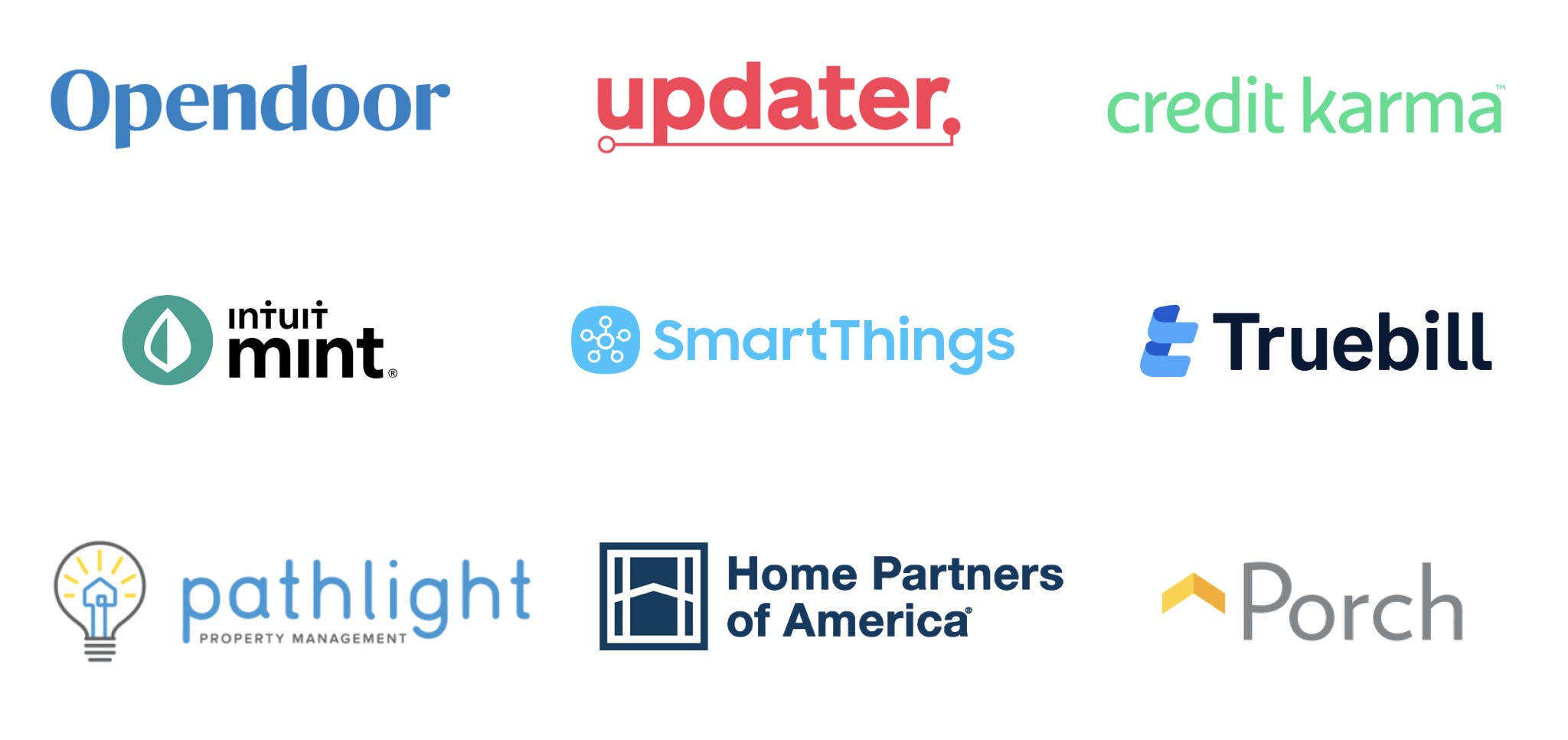The image features a white background showcasing the logos of nine different companies. 

1. **Open Door**: Positioned at the top left, the logo is presented in blue font.
2. **Updater**: Appears in red font, accompanied by a red line underneath and a red dot to the right, with a red outline dot containing a white center on the left.
3. **Credit Karma**: Displayed in light green font.
4. **Intuit Mint**: Located on the next line down to the left, in black font. It includes a green circle with a white mint leaf that has a touch of green inside.
5. **SmartThings**: Situated next to Intuit Mint, it features blue font and a logo of a blue circle with five blue circles around and a white outline circle inside.
6. **True Bill**: Presented in black font, alongside two curved strips in blue and darker blue.
7. **Pathlight**: On the left, this logo showcases a black outline of a light bulb filled with yellow lines and a blue house in the middle. The text reads "Pathlight" in blue, with "Property Management" in gray underneath.
8. **Home Partners of America**: Features a dark blue font and includes a blue outlined box with a broken image in blue within it.
9. **Porch**: The logo comprises a light yellow and orange arrow pointing up, with the word "Porch" in gray.